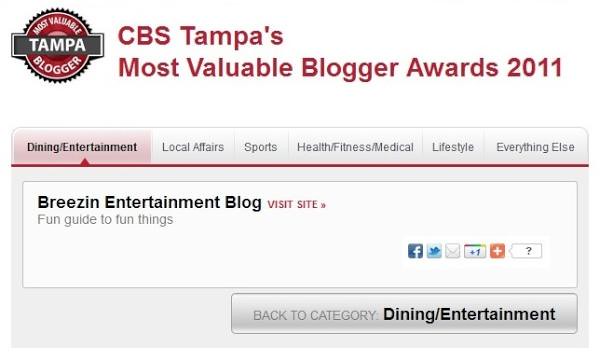The close-up image of a website showcases a predominantly white background with striking red and black text. Prominently featured in the upper left corner is a rounded logo with a red circle intersected by a gray bar. The logo reads "Most Valuable Tampa Blogger" — "Most Valuable" at the top in white font, "Blogger" at the bottom, and "Tampa" inside the central gray bar. Adjacent to the logo, large red text announces "CBS Tampa's Most Valuable Blogger Awards 2011." 

Below this prominent header is a series of clickable tabs within a gray box. The tab on the far left, highlighted in red, reads "Dining/Entertainment," indicating it has been selected. The tab's selection reveals a white text box beneath it, displaying "Breezen Entertainment Blog" in black font with a red "Visit Site" link. 

The lower right corner of the image features icons for social media platforms, such as Facebook and Twitter, along with options for email and more. At the very bottom of the image, a button provides the user the option to go back to the "Dining/Entertainment" category, ensuring easy navigation within the site.